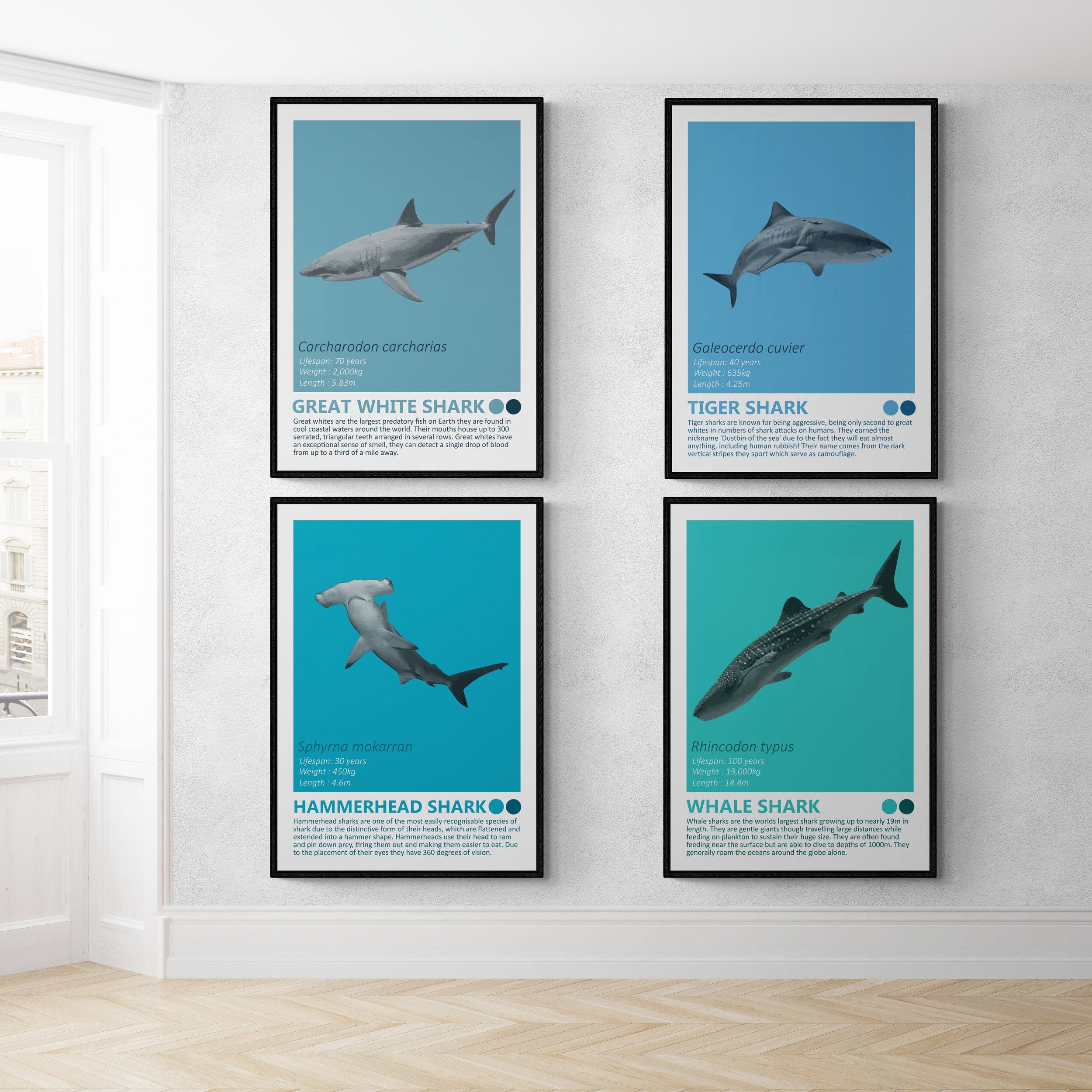This interior photo captures a room with white walls and white trim, featuring a laminate wood floor with a zigzag pattern. A window on the left offers a view of a brick exterior. The focal point of the image is a series of four large, framed pictures of different shark species, each displayed in sleek, narrow black frames. The sharks are arranged in a clockwise manner starting from the upper left: Great White Shark (Carcharodon carcharias), Tiger Shark (Galeocerdo cuvier), Whale Shark (Rhincodon typus), and Hammerhead Shark (Sphyrna mokarran).

Each frame contains not just the image of the shark but detailed information about the species. The Great White Shark frame notes that they are the largest predatory fish on Earth, found in cool coastal waters worldwide. This frame specifies their notable number of up to 300 serrated triangular teeth and an exceptional sense of smell.

The Tiger Shark frame highlights their aggressive nature and eclectic diet, earning them the nickname "dustbin of the sea." Their dark vertical stripes serve as camouflage.

The Hammerhead Shark frame describes their distinctive hammer-shaped head, which they use to trap prey, and their 360-degree vision due to their eye placement.

The Whale Shark frame presents them as gentle giants, the world’s largest sharks, often found feeding on plankton near the surface but capable of diving to depths of 1,000 meters.

The frames’ cohesive design, with light and dark blue color coding, along with some green hues for the Whale Shark, adds to the educational feel reminiscent of a museum display.